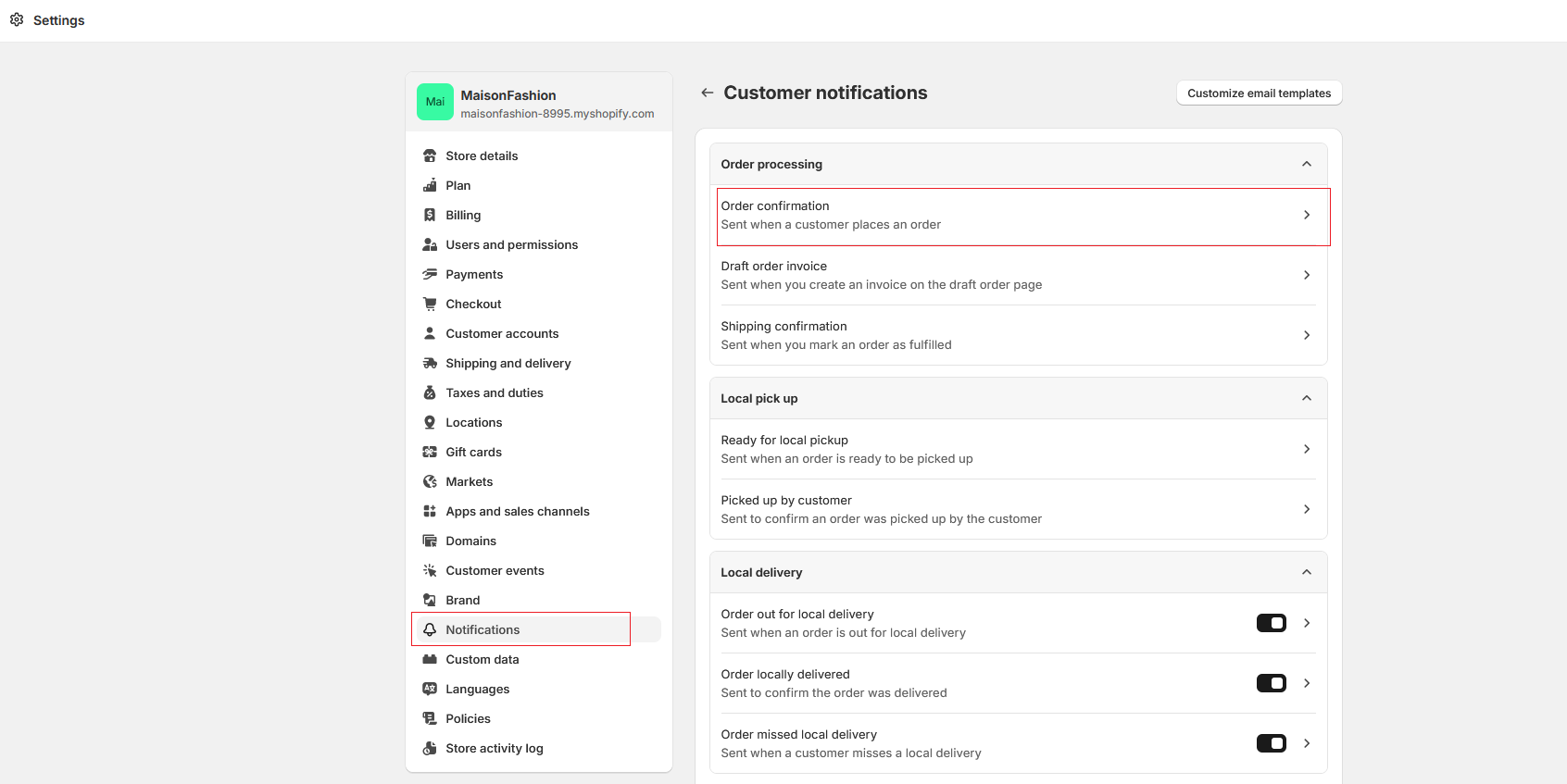Screenshot of an E-commerce Settings Panel

The image is a screenshot of the settings panel from an online shop's webpage, resembling a web storefront interface. At the top of the page, there is a title "Settings" in black font, accompanied by a cogwheel icon to the left.

The webpage features a gray background and has two central panels. On the left side, there is a small box designated for a profile picture, followed by the text "Maison Fashion" in bold black letters. Below this, there is an address that reads "dot my spotify.com". This left panel vertically lists several menu options: Store Details (with a store icon), Plan (with a bar graph icon), Billing, User Permissions, Payments, Checkout, Customer Accounts, and Notifications (with a notification bell icon). The Notifications option is distinctly highlighted with a red border.

On the right side of the panel, which is expanded, the heading "Customer Notifications" is displayed with a left-pointing arrow adjacent to it. The first category under this heading is "Order Processing". The initial option under Order Processing, titled "Order Confirmation," is specifically highlighted with a red border.

The screenshot effectively guides the viewer on selecting the Notifications option and subsequently clicking the Order Confirmation option under the Customer Notifications section.